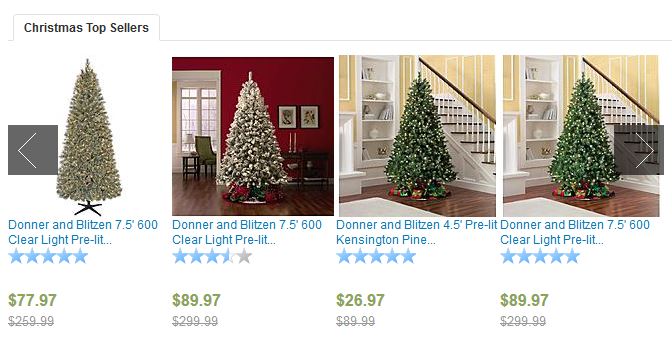The image showcases the top-selling Christmas trees online, featuring four distinct styles with updated prices, ratings, and decorations.

1. **Donner & Blitzen 7.5 ft Pre-lit Christmas Tree**: This tree features 600 clear lights, standing 7.5 feet tall. It has earned a perfect 5-star rating. Originally priced at $259.99, it is now available for $77.97.

2. **Donner & Blitzen 7.5 ft Pre-lit Christmas Tree**: Similar to the first, this tree also stands 7.5 feet tall and has 600 clear lights, but it has garnered a 3.5-star rating. Originally $299.99, it is currently priced at $89.97. The tree is displayed in an elegant room with a red wall backdrop and hardwood flooring.

3. **Donner & Blitzen 4.5 ft Pre-lit Kensington Pine**: This smaller tree stands 4.5 feet tall, featuring a lush Kensington Pine design. It has received a 5-star rating. The original price was $89.99, and it is now offered at $26.97. The setting includes a well-decorated room with hardwood floors, yellow walls, white stairs, and white furniture.

4. **Donner & Blitzen 7.5 ft Pre-lit Christmas Tree**: This tree, also 7.5 feet tall with 600 clear lights, has achieved a 5-star rating. Originally listed at $299.99, it is now available for $89.97. This tree is shown in the same beautifully decorated room as the previous image, featuring hardwood flooring, yellow walls, white stairs, and white furniture.